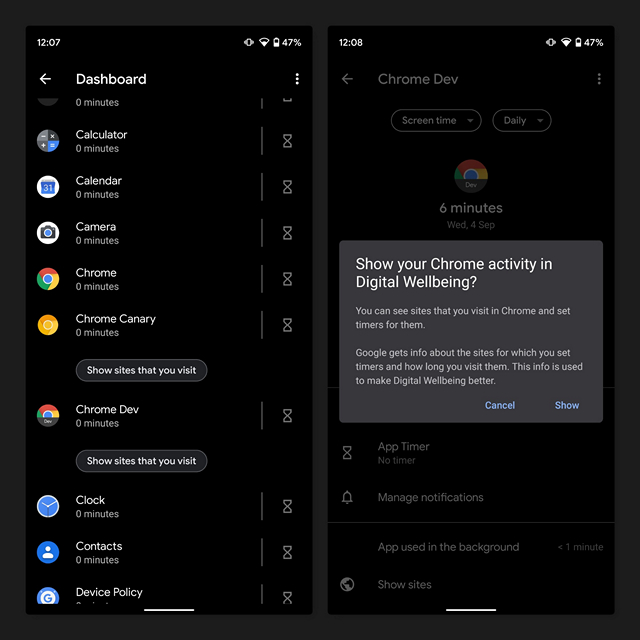**Detailed Caption:**

The image displays two side-by-side screens of a phone, both set against a black background. The left screen shows a time of 12:07, while the right screen reads 12:08. Both screens display a battery charge of 47%.

On the left screen, an arrow pointing left accompanies the word "Dashboard" at the top, with a list beneath it showing various apps and their usage times, all listed as "Zero Minutes." The apps include: "Calculator," "Calendar," "Camera," "Chrome," "Chrome Canary," "Chrome D.E.V," "Clock," and "Contact." There are two gray ovals within this list—each followed by the text "Show Sites That You Visit."

The right screen features an arrow pointing left at the top next to the title "Chrome Development." Below this, there are two ovals with text in white stating "Screen Time" and "Daily Run IC." It details usage information as "Six Minutes WED4SAP." A gray pop-up rectangle appears with a message in white: "Show Your Chrome Activity and Digital Wellbeing. You can see sites that you visit in Chrome and set timers for them. Google gives info about the sites for which you set timers and how long you visit them. This info is used to make digital wellbeing better." At the bottom of this pop-up, there are two buttons: "Cancel" in blue and "Show" in blue.